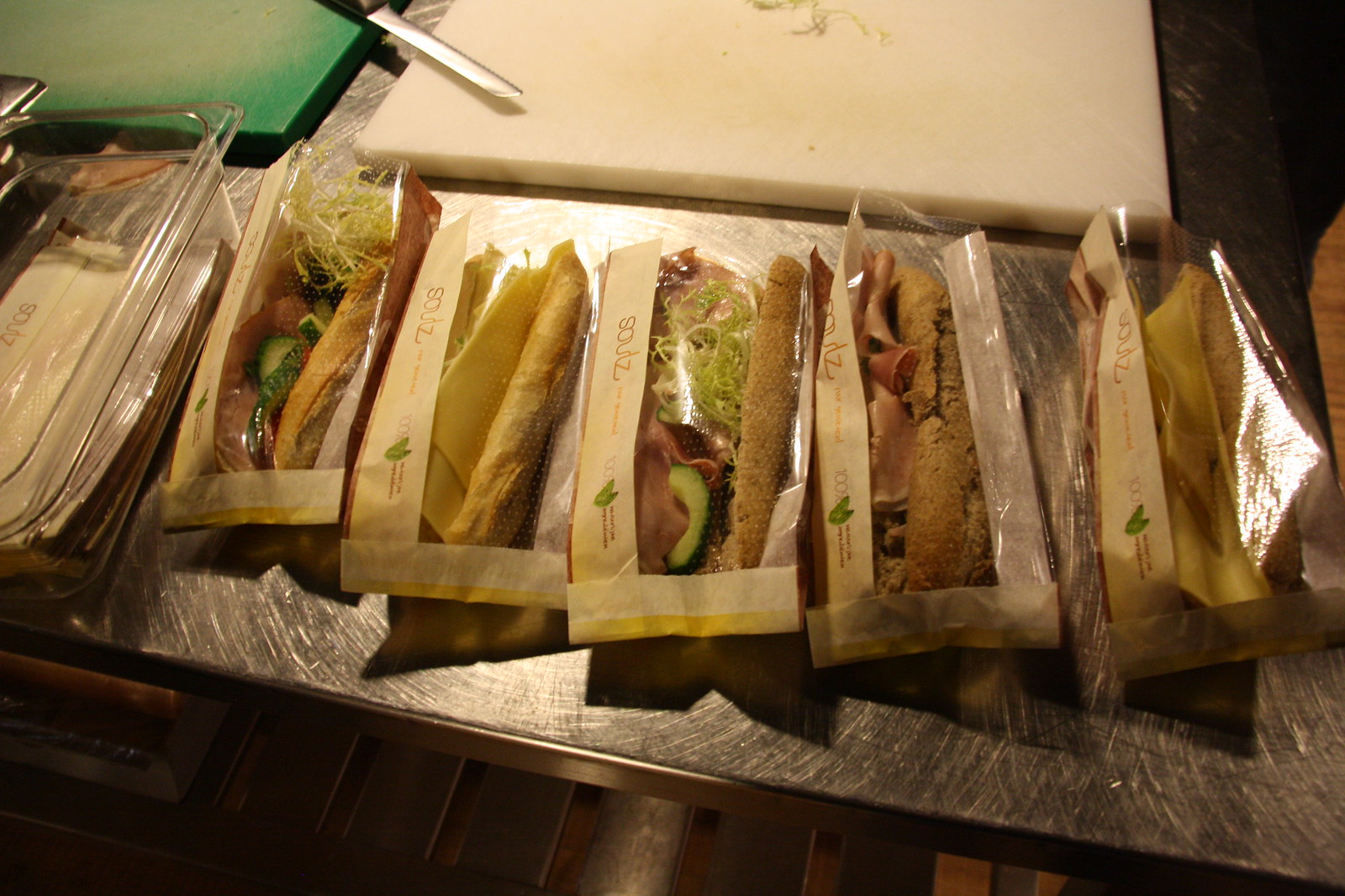This photograph showcases five sandwiches displayed on a scratched stainless steel countertop. The sandwiches, made on French or hoagie rolls, are contained within clear cellophane wrappers that reveal a variety of fillings including meats, vegetables like lettuce, cucumbers, and avocado, and some sliced cheese. Each sandwich packaging bears a brand name that appears to read "SOULZ" or "SOLZ," though it's slightly unclear. Positioned in front of the sandwiches is a white cutting board with remnants of food and a knife placed diagonally. To the left of the white cutting board, there is another green cutting board. Also visible to the very left is a clear plastic bin holding additional sandwich wrappers, ready for use.